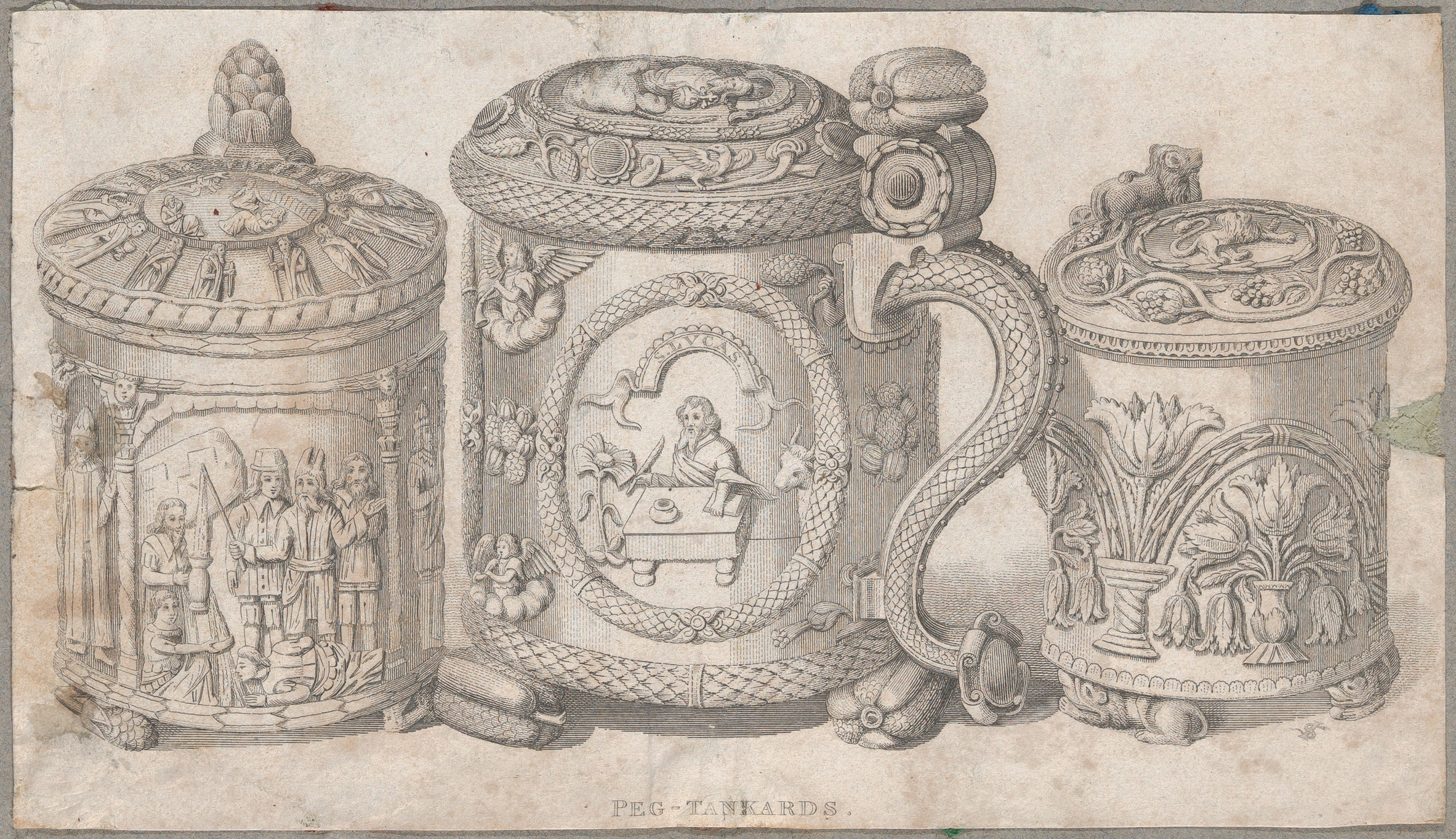This detailed pencil drawing in grayscale depicts three ornately decorated antique tankards labeled "peg tankards" at the bottom. The tankard on the left stands on feet and features decorative carvings of ancient-looking figures and Saints around the top. The lid is adorned with what appears to be an artichoke-like handle. The central tankard is the largest in both diameter and height with a dragon tail-shaped handle and rests on squash-shaped legs. It is richly embellished with rope-like embossing, a scene of a man seated at a desk surrounded by angels, and flowers around the base of the lid. The tankard on the right also stands on feet, with carvings of flowers and intricate grapevines. A thumb flip on each contributes to their practical design. The lid is topped with a figure that could be either a bear or a lion, adding to the tankard's elaborate detail. The surfaces of all three tankards are extensively detailed with hatch marks, showcasing a high level of craftsmanship in their engraved and carved designs.